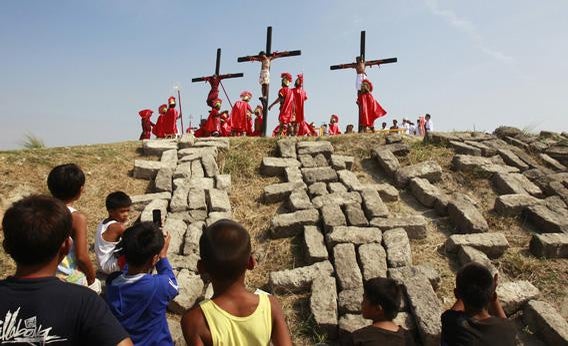In this detailed photograph, captured during the day against a light gray-blue sky, we observe a somber reenactment of the crucifixion of Christ. The setting is a grassy hillside scattered with chiseled rectangular stones or cement blocks. At the top of the hill, three wooden crosses stand with figures affixed to them—Jesus in the middle adorned with a small piece of white fabric, and two others on either side. Surrounding these crosses are Roman soldiers donning red helmets and flowing robes or capes, adding to the historical ambiance. In the foreground and to the sides of the hill, groups of children and a few adults gather to witness this poignant scene, their presence indicative of an educational or communal event. The meticulous arrangement and costumes contribute to a vivid, though somewhat distant, portrayal of this pivotal moment in history.